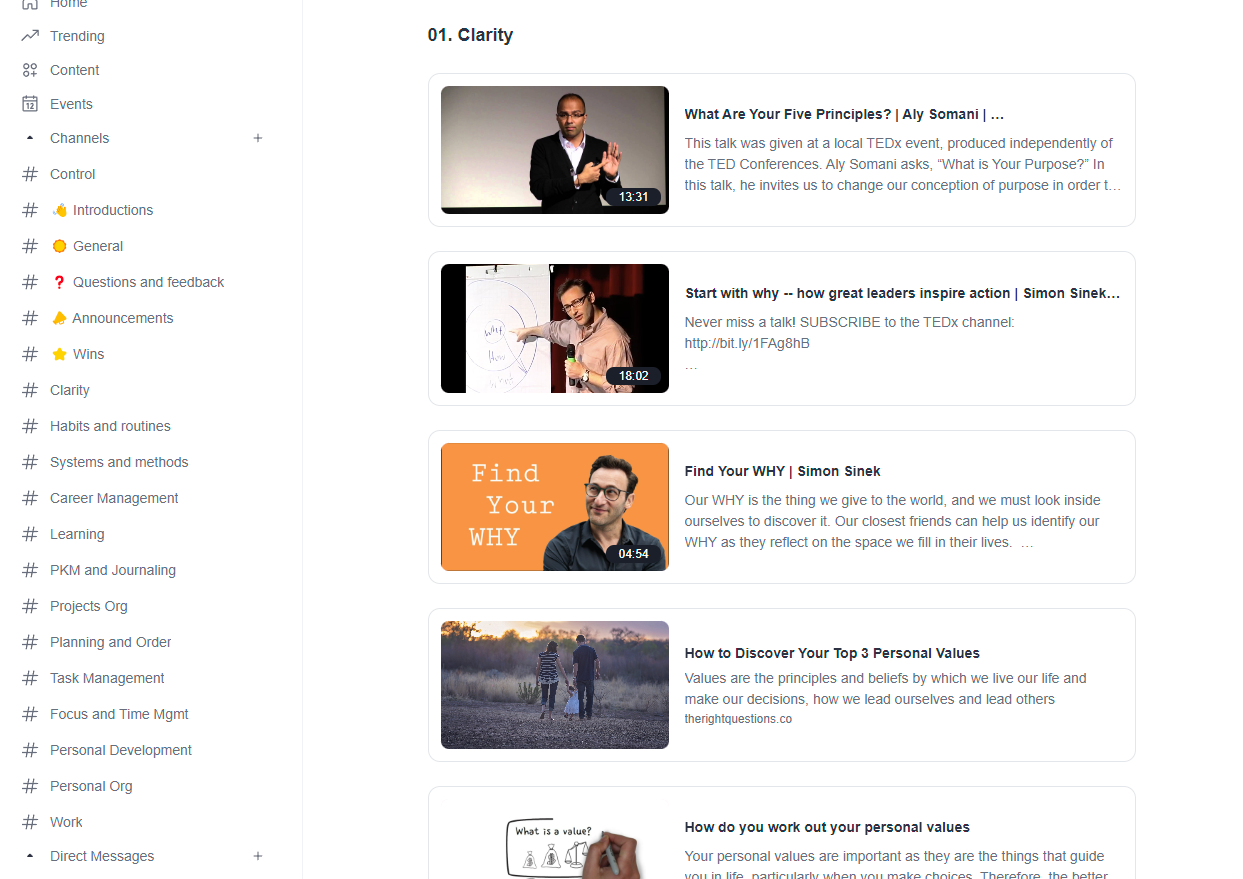This screenshot captures the home page of a website titled "Zero One Clarity." At the top of the page, the website's name "Zero One Clarity" is prominently displayed. Below the header, various entries resembling articles and videos are listed.

The first entry is titled "What Are Your Five Principles?" and features a video with a duration of 13 minutes and 30 seconds, which is a TED Talk.

The next entry is a video titled "Start with Why: How Great Leaders Inspire," with a length of 18 minutes. This is followed by another video, "Find Your Why" by Simon Sinek, which lasts 4 minutes and 54 seconds.

Below that is an article titled "How to Discover Your Top Five Personal Values." The final entry in the list is an article named "How Do You Work Out Your Personal Values?"

To the side of these entries, various hashtags categorize the content into topics such as "Control," "Introduction," "General Questions and Feedback," "Announcements," "Wins," "Clarity," "Habits and Routines," "Systems and Methods," "Career Management," "Learning," "PKM and Journaling," "Projects or Planning," "Task Management," "Focus and Time Management," "Personal Development," and "Personal or Work" under the category "Detect Messages."

This comprehensive home page offers a mix of videos and articles aimed at personal and professional development, categorized meticulously for easy navigation.